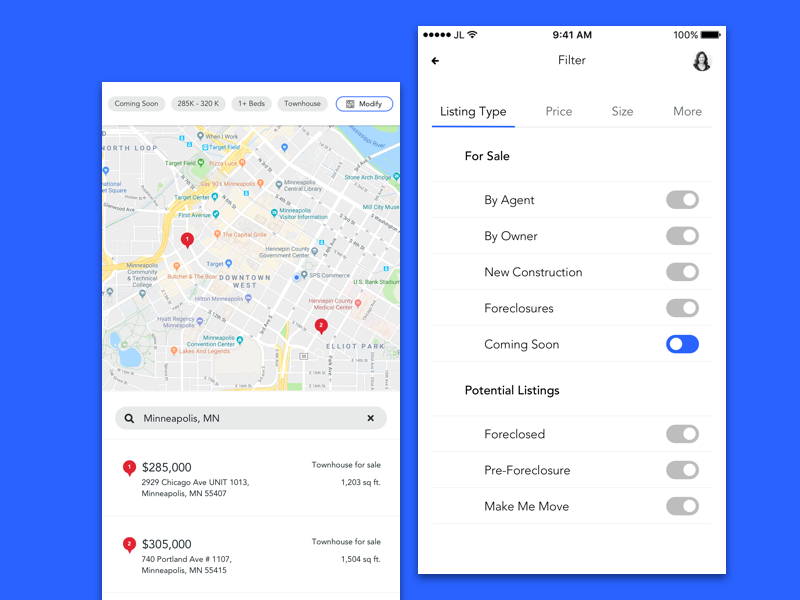This image showcases two screenshots from a smartphone, placed against a blue background. The first screenshot features a section of Google Maps displaying real estate listings in Minneapolis, Minnesota. At the top, there's an indication of price range: "$285,000 to $320,000" for "1+ beds townhouse," accompanied by a "modify" button in the search bar. Below the map, two markers numbered "1" and "2" are labeled in red. Marker one lists a price of "$285,000," including the unit's address, while marker two shows a price of "$305,000," along with its respective address.

The second screenshot, captured at 9:41 a.m., displays a real estate filter settings page. This page has four categories at the top: "Listing Type" (which is currently selected), "Price," "Size," and "More." Under the "Listing Type" section, the options available are "For Sale by Agent," "By Owner," "New Construction," "Foreclosures," and "Coming Soon," each accompanied by a toggle switch. Only the "Coming Soon" toggle switch is turned on. Below these, additional options include "Potential Listings," "Foreclosed," "Pre-Foreclosure," and "Make Me Move," all with their toggles switched off.